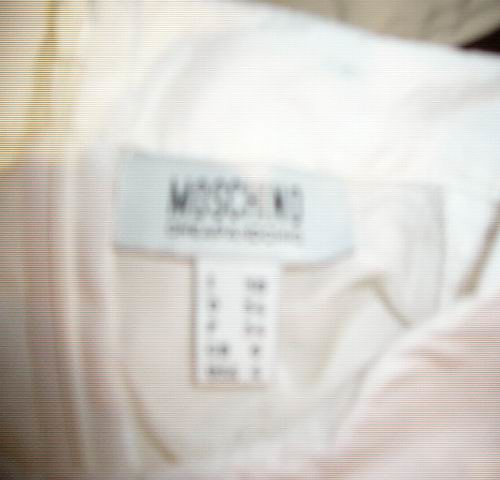This image is a highly zoomed-in and blurry close-up of a Moschino clothing tag on a shirt. The shirt appears to be pink and is laying on white, fluffy sheets. The main tag is rectangular, white, and displays the brand name "Moschino" in bold black letters, with some smaller, illegible text below it. Hanging from the middle of this tag is a smaller vertical tag, likely indicating the garment's size and different countries' sizing information. Horizontal lines, possibly from a video screen or digital artifacts, are visible across the top and bottom of the photo. The closer you get to the image, the blurrier it becomes, but leaning back reveals more details. The garment itself seems soft and may have ruffled or folded edges, adding to its indistinct, blurred presentation.